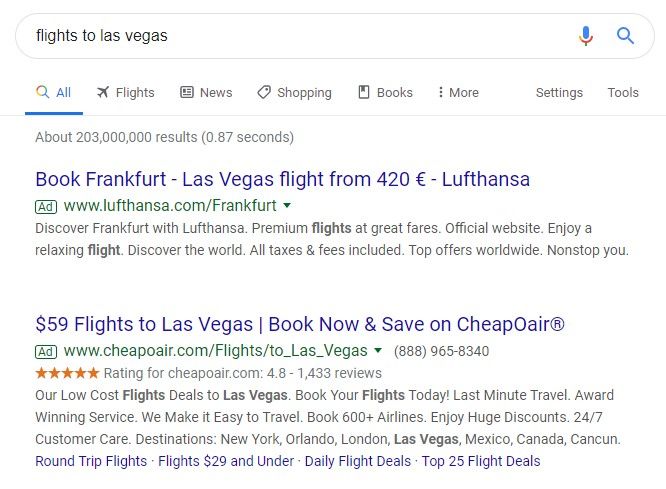The image depicts a Google search results page for "flights to Las Vegas." The layout is primarily white, featuring black and blue text. Notably, the first two visible results are advertisements:

1. The first ad offers a "Book Frankfurt to Las Vegas flight from €420" through Lufthansa. This link includes a brief description: "Discover Frankfurt with Lufthansa. Premium flights at great fares. Official website."

2. The second ad promotes "$59 flights to Las Vegas" via CheapOair, encouraging users to "Book now and save." The description reads: "Our low-cost flight deals to Las Vegas. Book your flights today. Last minute travel, etc."

Both advertisements are clearly marked with "Ad" next to them. Above these results, the search statistics indicate there are "about 203 million results" found in "0.87 seconds."

Additionally, the search bar is visible at the top of the page, complete with a microphone button for voice input. Just below the search bar, there are various tabs, including a "Flights" tab, to refine search results specifically related to flight information.